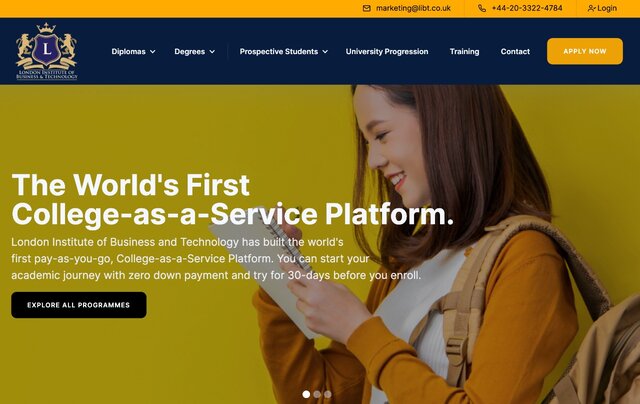The image is a screenshot of a website’s page displayed on a desktop interface, denoted by its layout. At the very top, there is a slim gold header featuring a login button in blue text located on the top right. Adjacent to the left of the login button, there is a phone number, and even further to the left, an email address formatted as marketing@something.co.uk.

Beneath this gold header is a much thicker dark blue header. On the far left of this header, a detailed crest logo is present, consisting of a purple shield with a gold border, a crown positioned above the shield, and two lions standing on either side with their forepaws resting on the shield. Adjacent to this logo, white text extends across the header listing several website sections: "Diplomas," "Degrees," "Prospective Students," "University Progression," "Training," and "Contact." On the extreme right of this thick header, a large orange rectangle with white text invites users to "Apply Now."

The body of the webpage has a mustard-colored background. Overlaid on this background is a photograph of a woman with long brown hair, wearing a brown long-sleeve shirt and a backpack slung over her shoulder. She is gazing towards the left, captured in profile. Superimposed upon this image is the bold declaration, “The world's first college as a service program.” Beneath this tagline is a short descriptive blurb, followed by a black rectangle with an invitation in white text that encourages visitors to “Explore All Programs.”